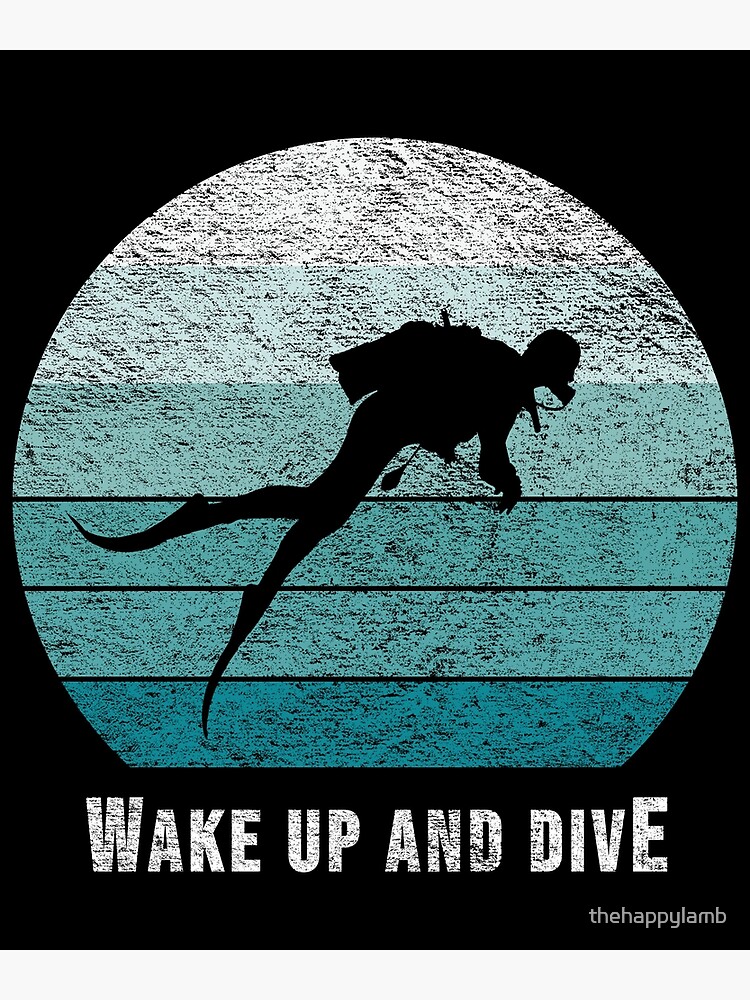The image features a logo set against a rustic wooden sign with a black border, centered around an oval-shaped, graduated blue area resembling planks on the side of a boat underwater. Within this blue section, there is a detailed silhouette of a deep-sea scuba diver equipped with an oxygen tank, mask, and flippers, creating the impression of looking through a telescope at the diver swimming alongside the submerged portion of a ship. The background of the image is segmented into layers of white, light blue, and dark blue, with specks of black adding texture. Below the diver silhouette, white text reads, "Wake Up and Dive," with smaller text beneath stating, "The Happy Lamb." The overall composition suggests an attractive, possibly promotional art print for a diving company.